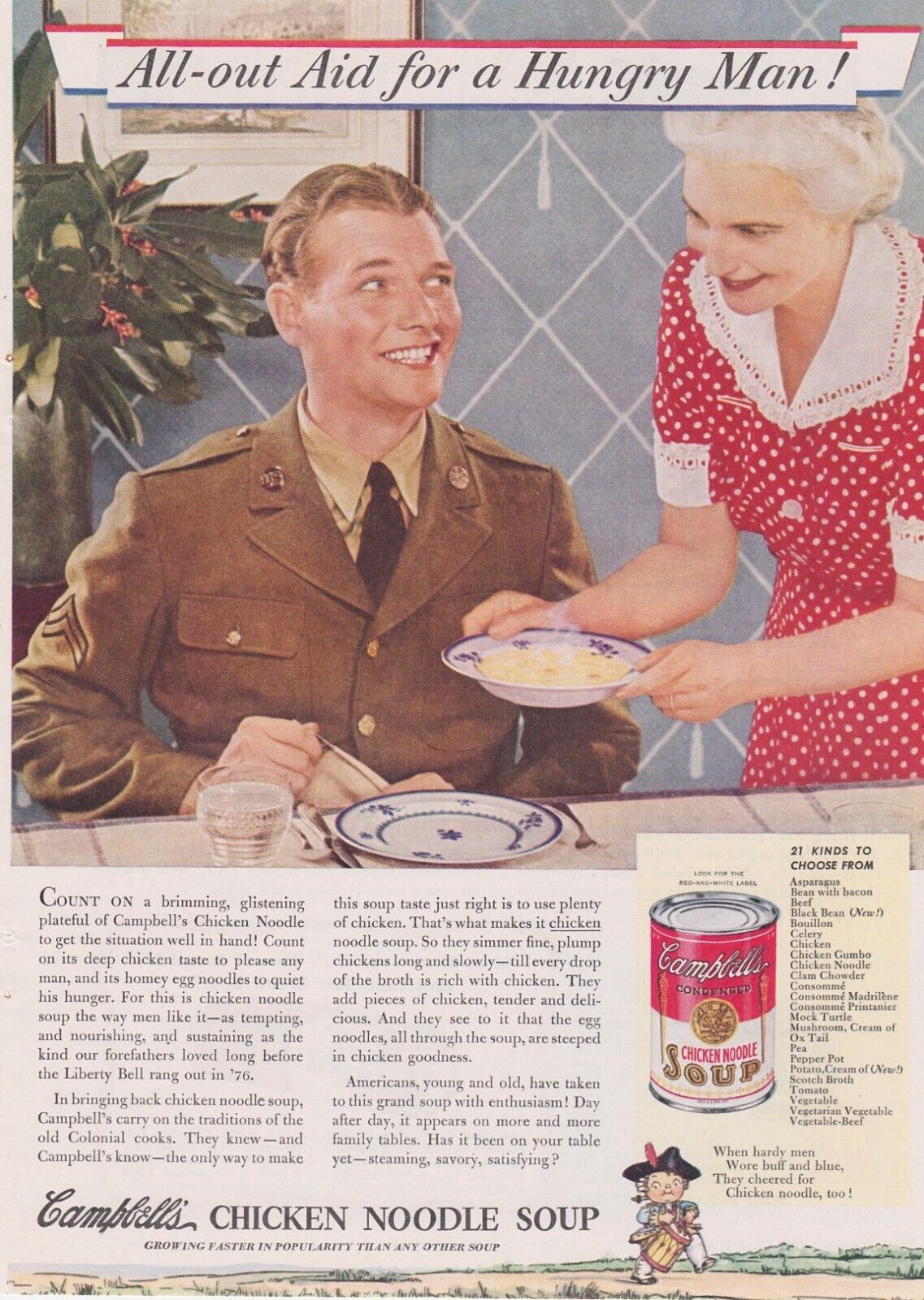In a nostalgic, vintage advertisement reminiscent of a Norman Rockwell painting, an Army soldier, likely home on leave, sits at a kitchen table, warmly smiling at an elderly woman serving him a steaming bowl of Campbell's Condensed Chicken Noodle Soup. The soldier wears a distinctive brown Army jacket adorned with epaulets, a tan collar, and a dark brown tie, while his cheeks blush with a vibrant, warm red hue. His short hair complements his green undershirt. Beside him, the elderly woman, presumably his mother, stands to his right wearing a red dress with white polka dots and white accents around the collar and sleeves. She holds a blue bowl with a white plate beneath it, both decorated with blue designs, and the creamy-colored soup inside steams invitingly.

In the background, the gray wallpaper with light gray diamond patterns adds a homely touch, complemented by a small plant and a framed picture. Above them, a prominent red, white, and blue ribbon banner reads, "All Out Aid for a Hungry Man." Below this, two paragraphs extoll the virtues of Campbell's Soup. To the right, the iconic Campbell’s Soup can displays its familiar branding with "Campbell's" in white, "Chicken Noodle" in red, and "Soup" in black and yellow. At the very bottom of the ad, against a backdrop of tan dirt and green grass, a man in a blue uniform with white shoes and a black hat adorned with blue and red feathers marches while playing a drum, adding a whimsical, patriotic touch to this classic, heartfelt scene.